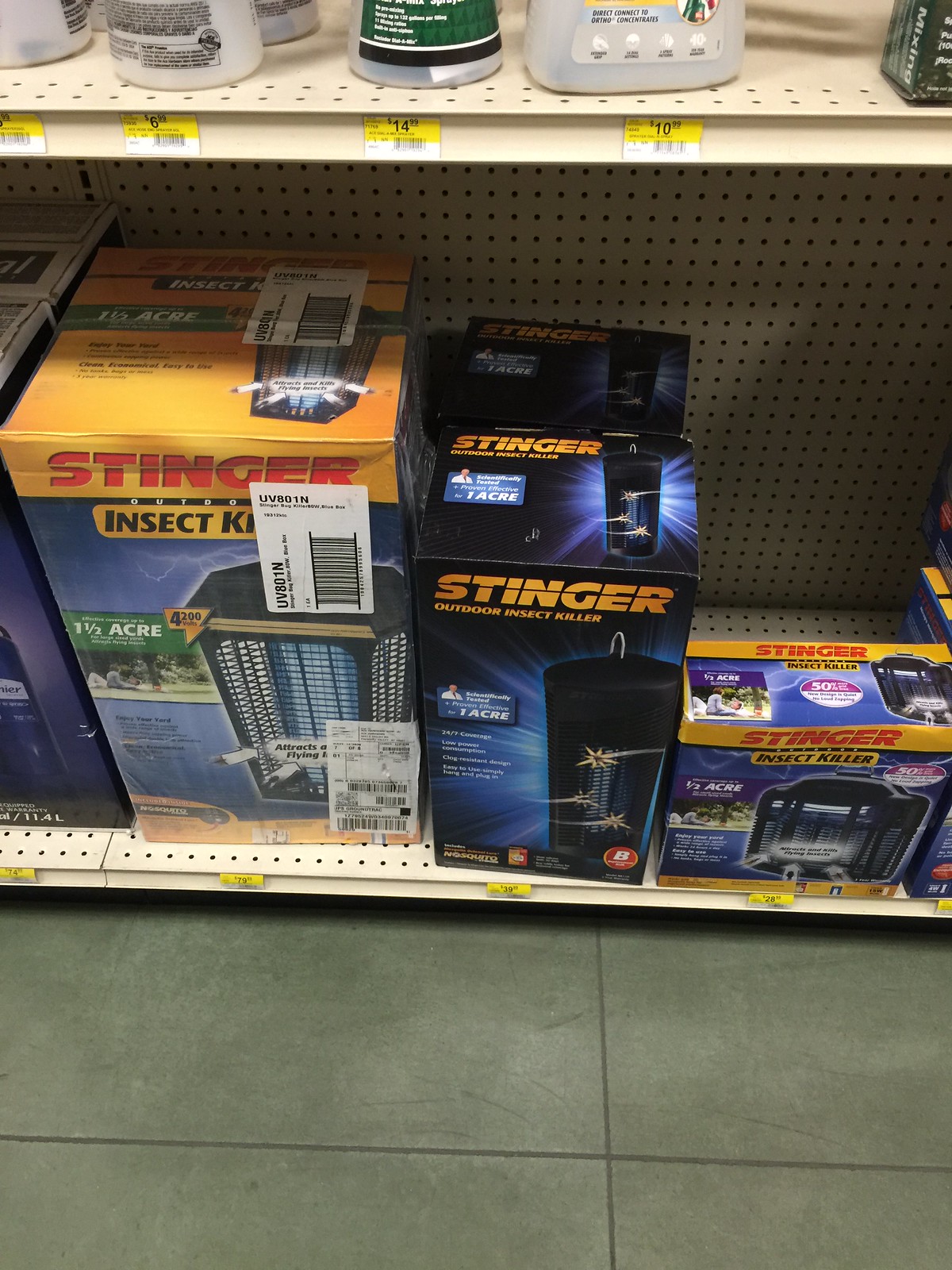This vertically aligned rectangular photograph captures a shelf display from a home improvement store, likely Home Depot, featuring various insect killer products. The beige-colored shelves, perforated with small circular dots, are mounted above a medium dark gray tile floor interspersed with lighter gray hues and gray grout lines.

On the bottom shelf, three boxes of Stinger insect killers are prominently displayed. The first box on the left, partially obscured by a barcode label, reads "Stinger Insect Kit" in white letters. Adjacent to it on the right is a box designed differently but also branded "Stinger." Further right sits a smaller box labeled "Stinger Insect Killer." These boxes predominantly feature blue and black colors accented with some yellow trim, along with black and red text.

The top shelf also holds insect-killing products, this time in plastic spray bottles with visible yellow and white price tags of $6.99, $4.99, and $10.99. Only the lower portions of the bottles are visible: two clear bottles on the left, one with a green and black label in the middle, and another clear bottle on the right.

In summary, the image portrays an organized display of insect killer products, emphasizing the Stinger brand, set against the neutral tones of the store's shelving and flooring.